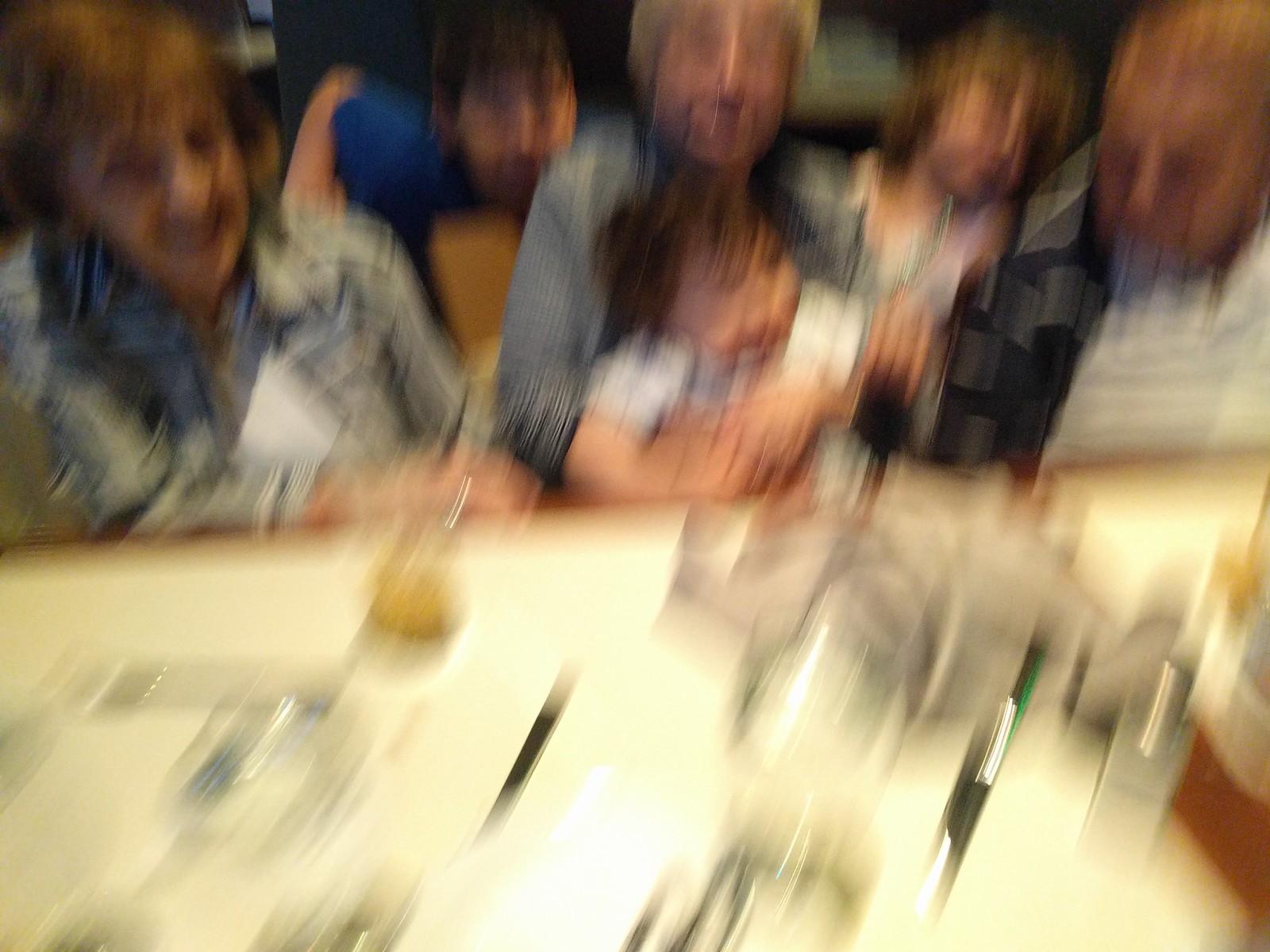An extremely blurry image shows a group of people seated at what appears to be a table. The table is in the foreground under a light that creates a slightly yellow hue on the surface, on which indistinct items, possibly bottles with silver lids and glasses with lemons, are scattered. In the background, which takes up the top half of the photo, we can make out three adults and a few children, though their features are obscured due to significant motion blur, likely caused by camera shake. An older lady sits on the far left, with a woman in the center holding a child with a white t-shirt. A man in a gray shirt sits on the right. In the back, a man in a blue shirt is visible between others. Another man, dressed in a white shirt with a gray and black checkered overshirt, also holds a child. Though the exact identities and relationships of the people are unclear, they might be a family gathering, captured in this snapshot of chaotic movement.